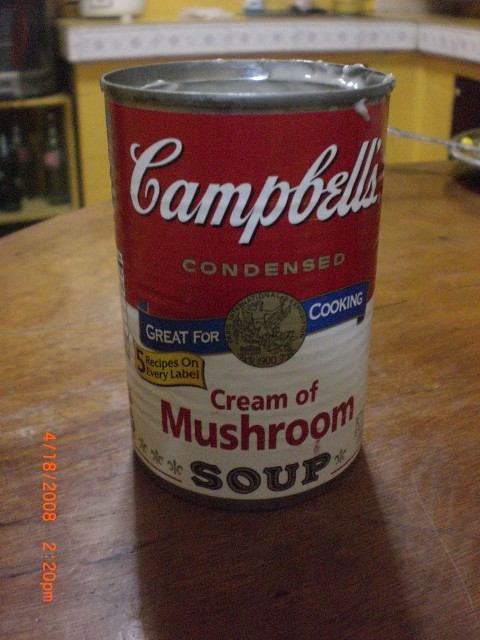This photograph captures a classic Campbell's soup can positioned prominently on a brown wood-grain table. The can, cylindrical and metallic, features the recognizable red and white label of Campbell's iconic design. The upper red section of the label bears the word "Campbell's" in white text, followed by "Condensed" in elegant gold text. The lower white portion of the label displays the variety "Cream of Mushroom" in vivid red text and "Soup" beneath it in black text. Adorning the center of the label is a bronze seal, flanked by blue ribbons, with the words "Great For" on the left and "Cooking" on the right. Just below the right ribbon, there is a gold background featuring the text "Five recipes on every label" in black lettering. The image background, slightly out of focus, reveals yellow kitchen cupboards, drawing attention solely to the can, which dominates the majority of the image.